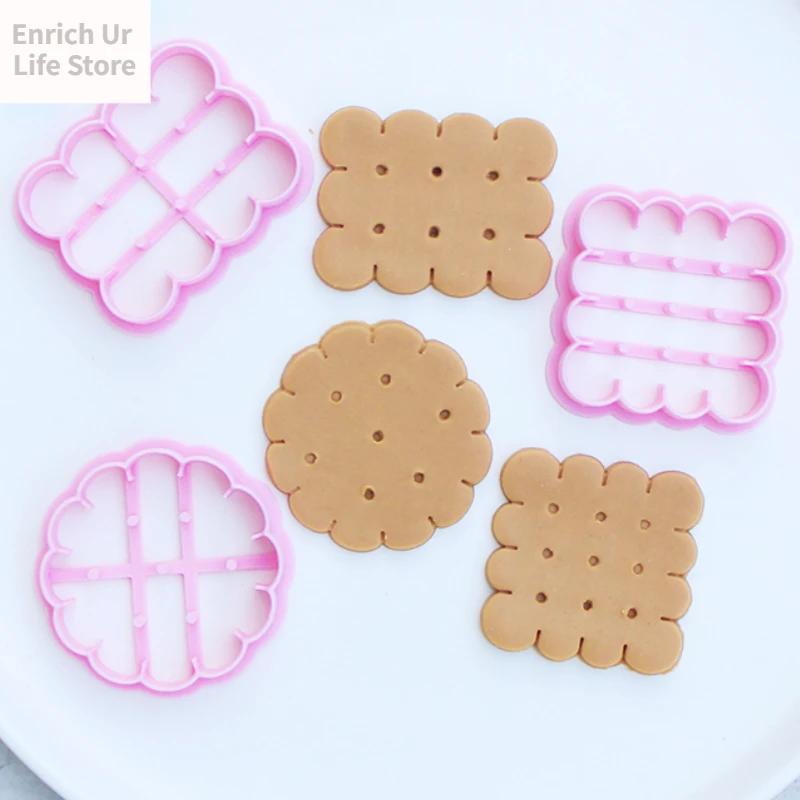The image showcases three pale pink cookie cutters and their corresponding unbaked cookie dough cutouts. In the top left corner, a gray font on a white rectangle reads "enrich your life store," with "year" uniquely spelled as "U R." The cookie cutters, positioned face up, include two with rounded, squarish shapes reminiscent of Biscoff cookie molds, and one with a circular, flower-like pattern featuring multiple petals and dot accents at the center. Each cutter is paired with a light brown cookie dough cutout placed adjacent to it, highlighting the shapes they create. The entire scene is set against what appears to be a white plate, visible at the bottom edge of the image.